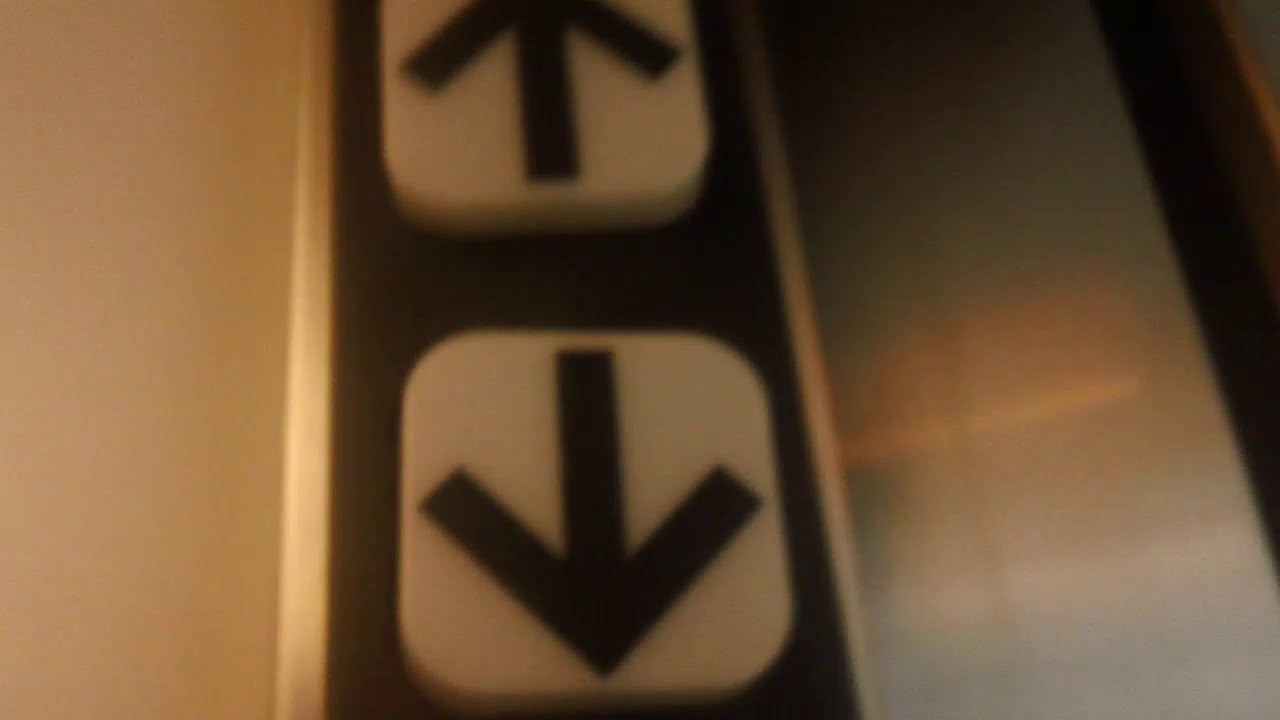The image depicts a slightly unfocused photo of an elevator call panel. Central to the image are two white rectangular buttons, each featuring black arrows indicating up and down directions. The top arrow is partially cut off at the top edge of the picture, while the bottom arrow is fully visible and more prominent. These buttons are set within a darker black frame. To the left of the buttons, there is a white surface, likely a wall. To the right, a stainless steel or metallic surface is visible, possibly part of the elevator door. In the far right corner of the image, there is a faint bluish-gray hue. The overall scene suggests a functional but unrefined capture of an elevator control panel, possibly within a building with multiple floors.